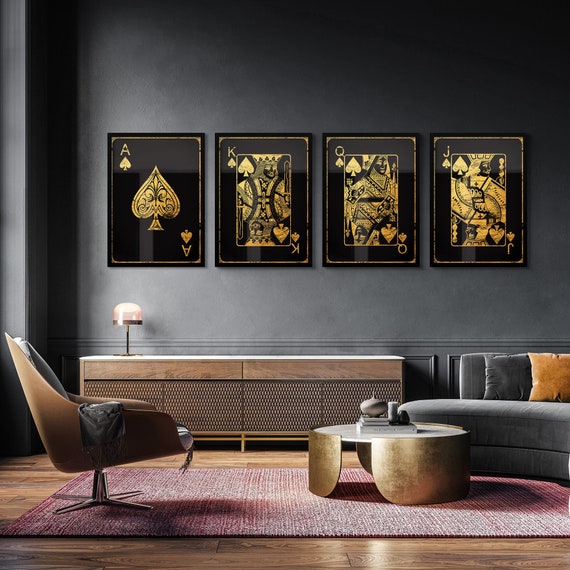The image depicts a stylish living room centered around four framed playing card illustrations, each featuring black cards with gold designs. From left to right, the cards are the Ace, King, Queen, and Jack of Spades, each detailed with gold borders, symbols, and lettering. The muted blue walls provide a sophisticated backdrop that complements a matching sofa positioned to the right. A round, gold-metal coffee table with large, decorative legs is prominently situated in front of the sofa. A pink rug adds a splash of color atop the hardwood floor. To the left, a chair reminiscent of an Eames lounge chair balances the room's aesthetic. Against the far wall stands a wooden cabinet with a white top, adorned by a small dome lamp on the left side. This eclectic combination of modern and classic elements creates a visually appealing and well-appointed living space.